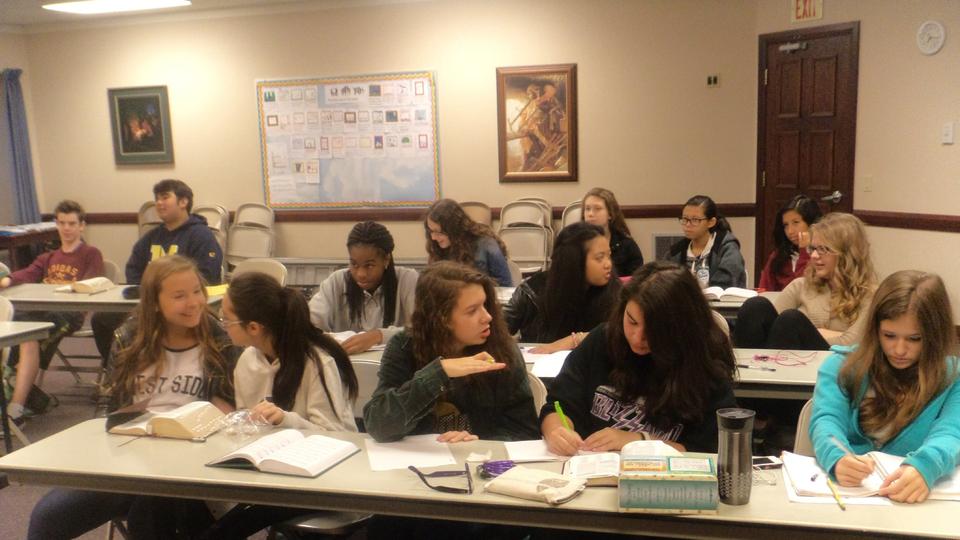The photograph captures an indoor classroom setting, filled predominantly with middle school or high school students. The classrooms feature large white desks arranged in rows. On the right-hand side, there are three tables, while the left side houses two additional tables. 

The front row prominently features five teenage girls, all appearing to be white. On the extreme left, a girl wearing an “Eastside” shirt is smiling at a girl to her right who has black hair, glasses, and is reaching into a plastic bag while an open book sits in front of her. Next to her is a white girl with long brown hair in a brown shirt. Another girl with an off-white sweatshirt, brown shirt, and purple keychain is looking towards a girl with black hair and a black t-shirt displaying something like the text “BLZZ.” This girl is diligently writing with a pen in her right hand among her books, including one open and one closed, beside which is a thermos or travel cup. The farthest right in the row is another white girl, with brown hair and a blue sweater, holding a pen.

Behind them, the next table has three girls: a black woman, a black girl with long hair and a gray shirt focused on her book, and a black girl wearing a black outfit and bracelet, who is glancing towards a blonde girl wearing glasses and a brown sweater.

In the third row at the last table on the right are several students, such as a white woman, a white girl in a red shirt, an Asian girl in a black sweatshirt, a white girl with a black shirt and brown hair, and another white girl with glasses and a gray sweater.

On the left side of the room, there is a partially visible table occupied by a boy in a red sweatshirt sitting next to an Asian boy in a black sweatshirt with the letter “M” on it. The boy in red is wearing shorts. Another table, barely within the frame, houses two more male students whose details are indistinct.

In the background, the classroom decor includes a blue and white blackboard, flanked by portraits on either side - one of a woman and another that appears to be a painting or print of a fire, with a map in between. The upper-right corner of the image shows a brown door marked with the word “Exit,” and to its right is a white wall clock.